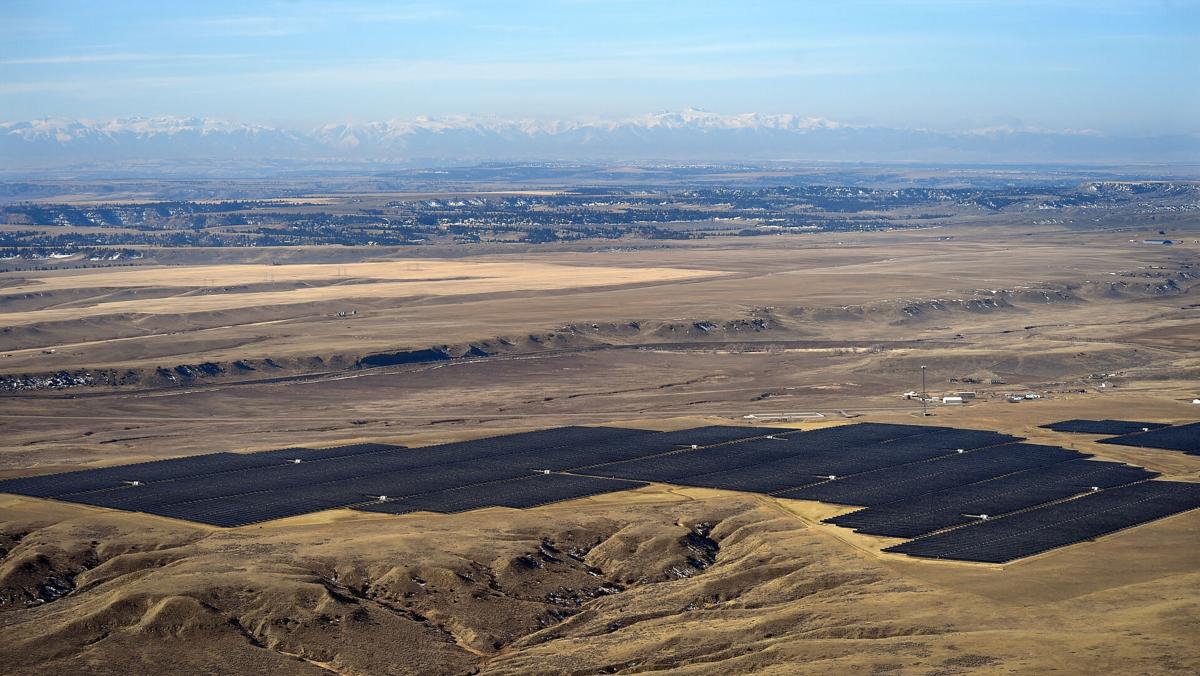This aerial photograph, likely taken from a plane or balloon, captures a vast, barren desert landscape stretching into the distance. In the foreground, the brown, empty land features several intentionally made squares, possibly agricultural fields, with more rectangles interspersed across the terrain, creating a patchwork effect. The ground is largely flat with subtle hills, and no distinct foliage or buildings are immediately visible. Further into the midground, the desert appears more expansive, dotted with a few scattered buildings and a road. Beyond these sparse developments lies a small mountain range with snow-capped peaks, giving way to an expansive backdrop of blue sky and clouds. This vast barren land extends all the way to the horizon, where a distant line of snow-capped mountains fades into the light blue sky, culminating in a blend of natural desolation and subtle human intervention.